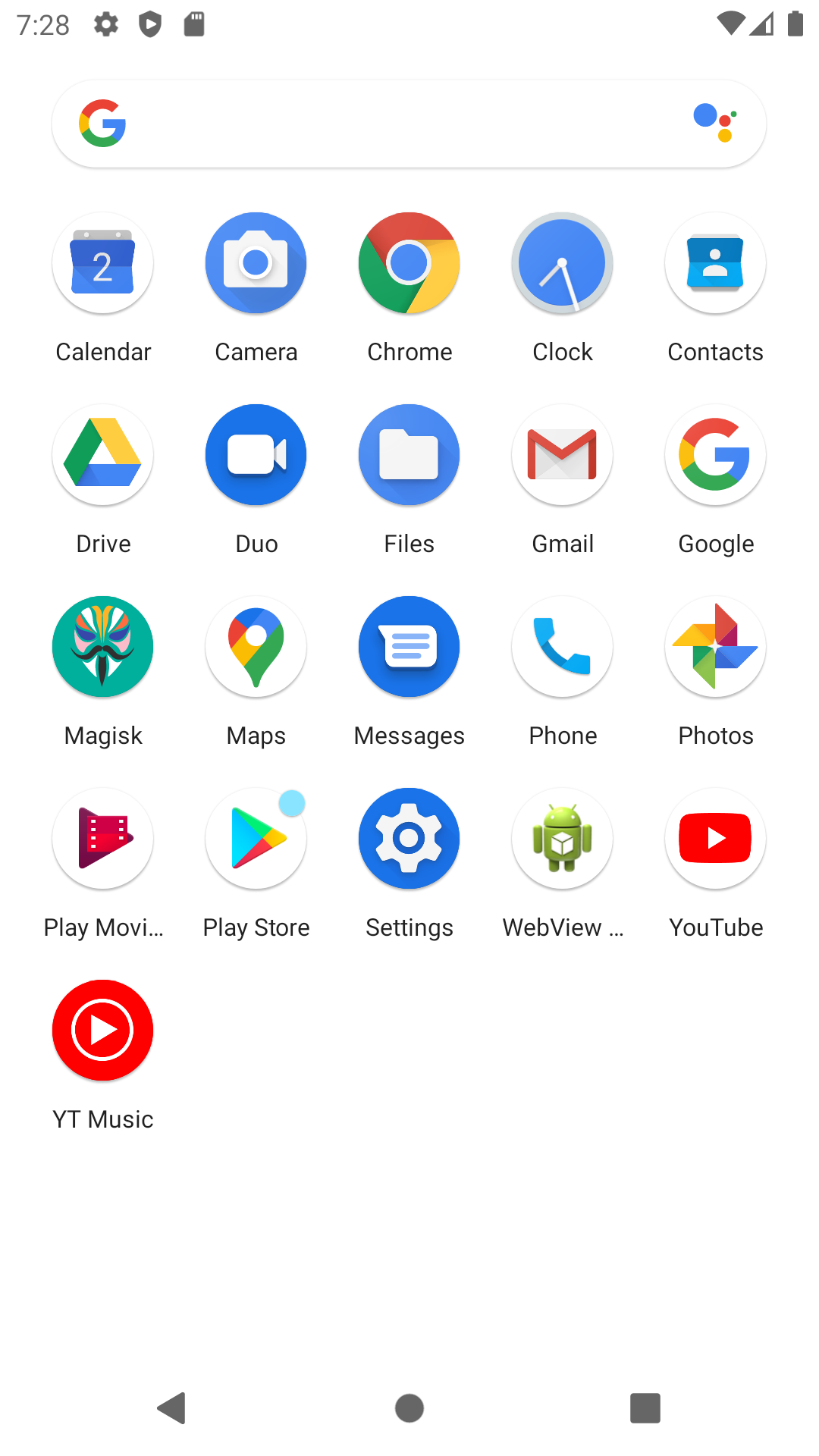A detailed screenshot of an Android tablet home screen is displayed, suggesting it might also be a larger phablet. The time reads 7:28, and the status bar indicates full Wi-Fi signal, approximately 75% cellular signal, and a fully charged battery. The Google search bar is visible at the top, empty and ready for input. Below the search bar, the home screen is organized with various app icons, totaling 21 in number, arranged in rows of five, except for the last row. 

From left to right, the icons are:
1. **Calendar** - displaying the date “2.”
2. **Camera** - represented by a white camera icon on a blue background.
3. **Chrome** - the multicolored circle with red, yellow, green, and blue segments.
4. **Clock** - a blue clock face with silver hands and rim.
5. **Contacts** - a white figure on a blue background.
6. **Drive** - a multicolored triangle in yellow, blue, and green.
7. **Duo** - a white classic webcam icon on a blue background.
8. **Files** - a white file icon on a blue background.
9. **Gmail** - a white envelope with a red outline.
10. **Google** - the recognizable multicolored 'G.'
11. **Magisk** - resembling a stylized Guy Fawkes mask with drag-style makeup.
12. **Maps** - a location pin in Google’s colors.
13. **Messages** - a white speech bubble on a blue background.
14. **Phone** - a blue phone icon on a white background.
15. **Photos** - a multicolored pinwheel-like icon.
16. **Play Movies & TV** - represented by a red film strip with the Play logo.
17. **Play Store** - the multicolored triangle pointing to the right.
18. **Settings** - a white cogwheel on a blue background.
19. **WebView** - partially cut off, displaying the Android robot with a white box.
20. **YouTube** - a red square with a white play button.
21. **YouTube Music** - a red circular target with a white play symbol. 

Overall, the screenshot provides a clear and organized view of the user’s main applications and configurations on an Android tablet.